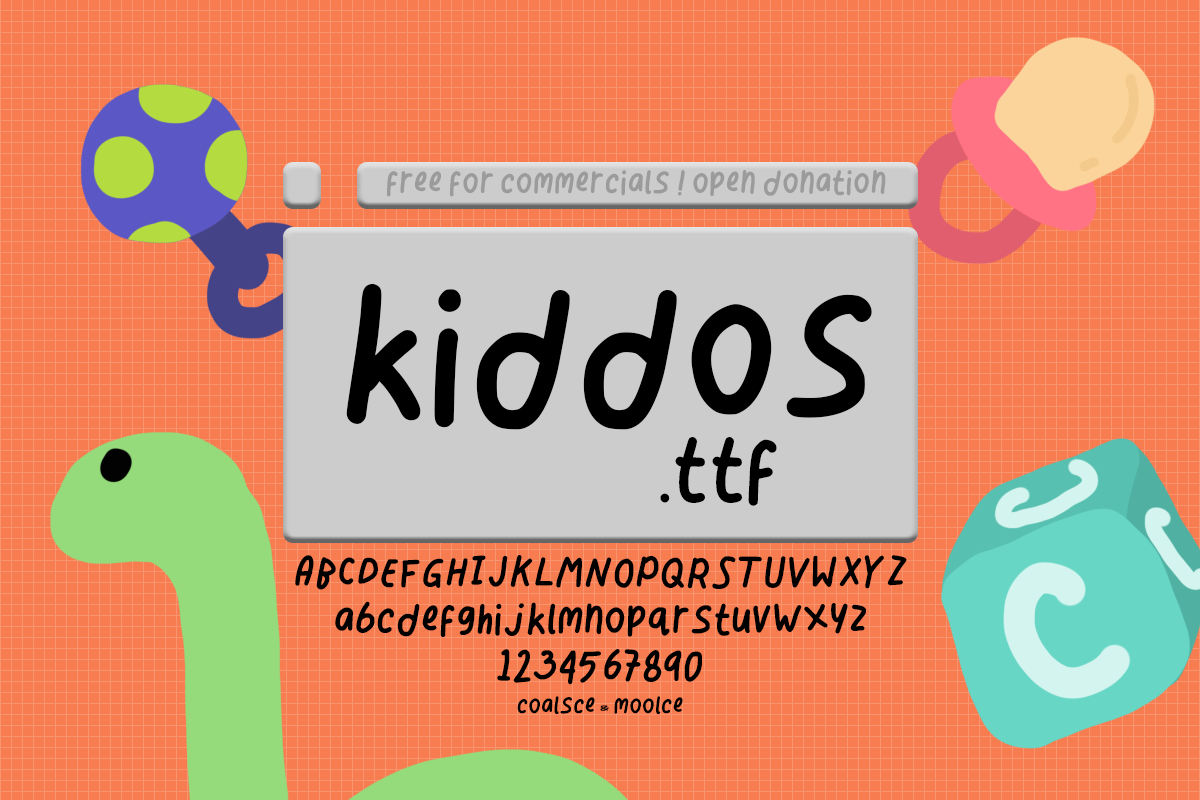The image features an orange background with a white grid overlay. Dominating the center of the image is a dark gray rectangle displaying text in the ‘Kiddos’ font, specifically 'kiddos.ttf'. Within this rectangle, there seems to be a passage written in an informal, playful style. 

Adjacent to this primary rectangle, there's a variety of colorful children's illustrations and toys. This includes a pink rattle with a blue handle decorated with green circles, a green dinosaur, and a blue cube labeled with the letter 'C' in white on each of its sides. Surrounding these items, there is a hand-drawn alphabet set, displaying all capital and lowercase letters from A to Z, along with numbers one through nine and zero.

Further details include a seemingly random combination of letters and words: "cols," "c-o-a-l-s-c-e," "m-o-o-i-c-e," and "louise m-o-o-i-c-e." 

At the top of the image, another dark gray rectangle bears the message: "Free for commercials! Open donation."